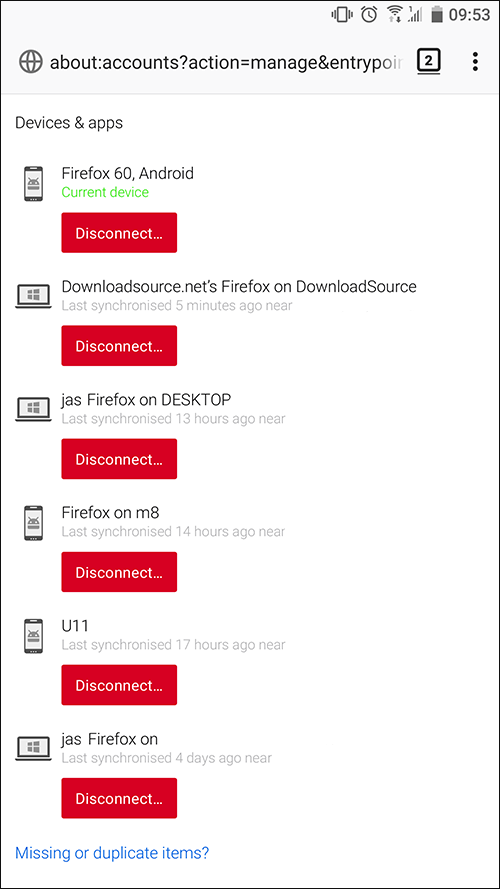The image is a screen capture taken from a digital device, displaying a screen with a predominantly white background. In the upper right corner of the screen, various icons are visible, including the battery icon and the time, which reads 9:53. Below the time, there is an internet icon—a round globe. To the right of this icon is a string of text that appears to be part of a search query or command: "about:accounts?action=manage&entrypoint".

In the main portion of the screen, written in dark gray on the left side, the text reads "Devices and Apps." Below this heading, the screen lists various apps and devices that are available for management. There are a total of six entries displayed. Each entry includes the name of a device or app written in green. Adjacent to each name, there is a red button. Each of these six red buttons bears the label "Disconnect" in white text.